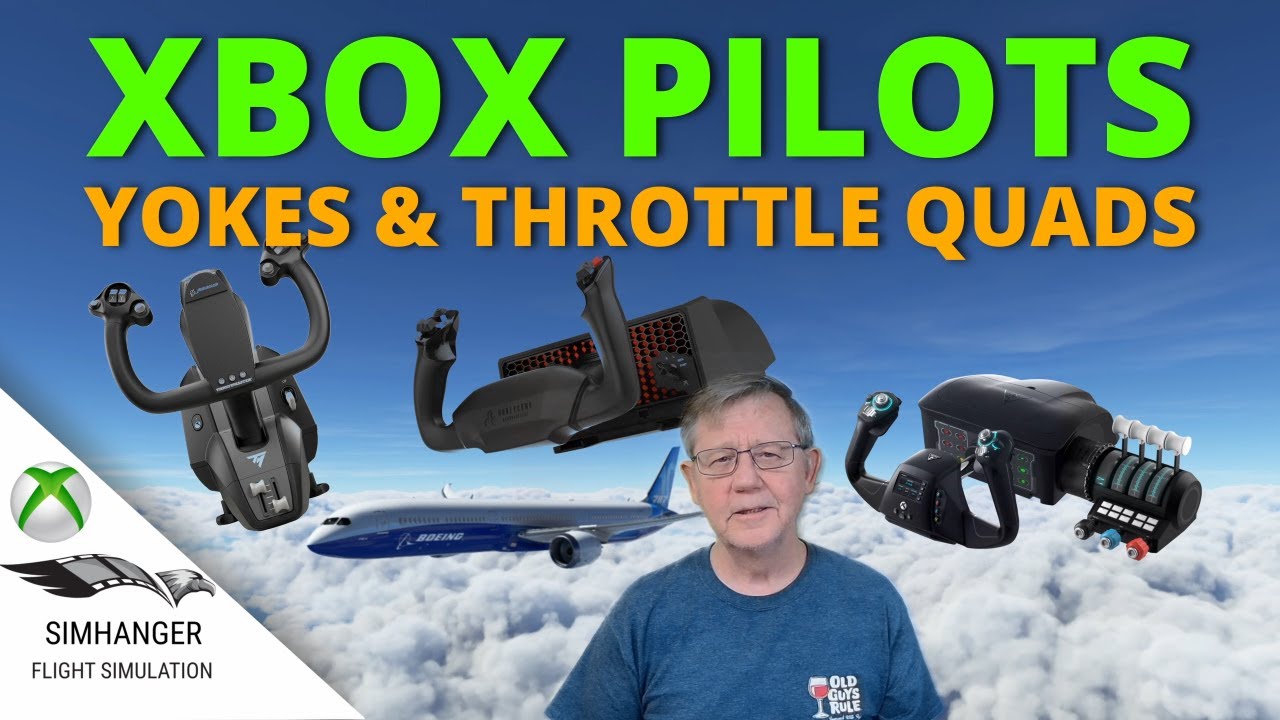The image is an advertisement showcasing flight simulation equipment endorsed by Xbox. Dominating the top of the ad, the words "Xbox Pilots" are written in a striking, boxy neon green font, while directly below it, a smaller orange text reads "Yokes and Throttle Quads." Below this, there are three distinct flight simulation yokes, depicted in black and appearing as if they're floating midair.

The left and right yokes are positioned symmetrically, with a third, more detailed yoke on the far right featuring additional speed handles and small knobs in black, red, and blue colors. Positioned beneath the first two yokes, a sleek Boeing aircraft is shown soaring above a sky filled with thick, fluffy clouds, contrasting with the clear azure backdrop.

On the left side of the image, an Xbox logo prominently displayed, just above black lettering that reads "Sim Hangar Flight Simulation," which includes a stylized green "X" on a white sphere and an emblem resembling a film roll wing with an eagle head.

In the foreground stands an elderly man with salt-and-pepper hair and glasses, wearing a blue t-shirt. The shirt features the phrase "Old Guys Rule" accompanied by a wine glass icon filled with red wine.